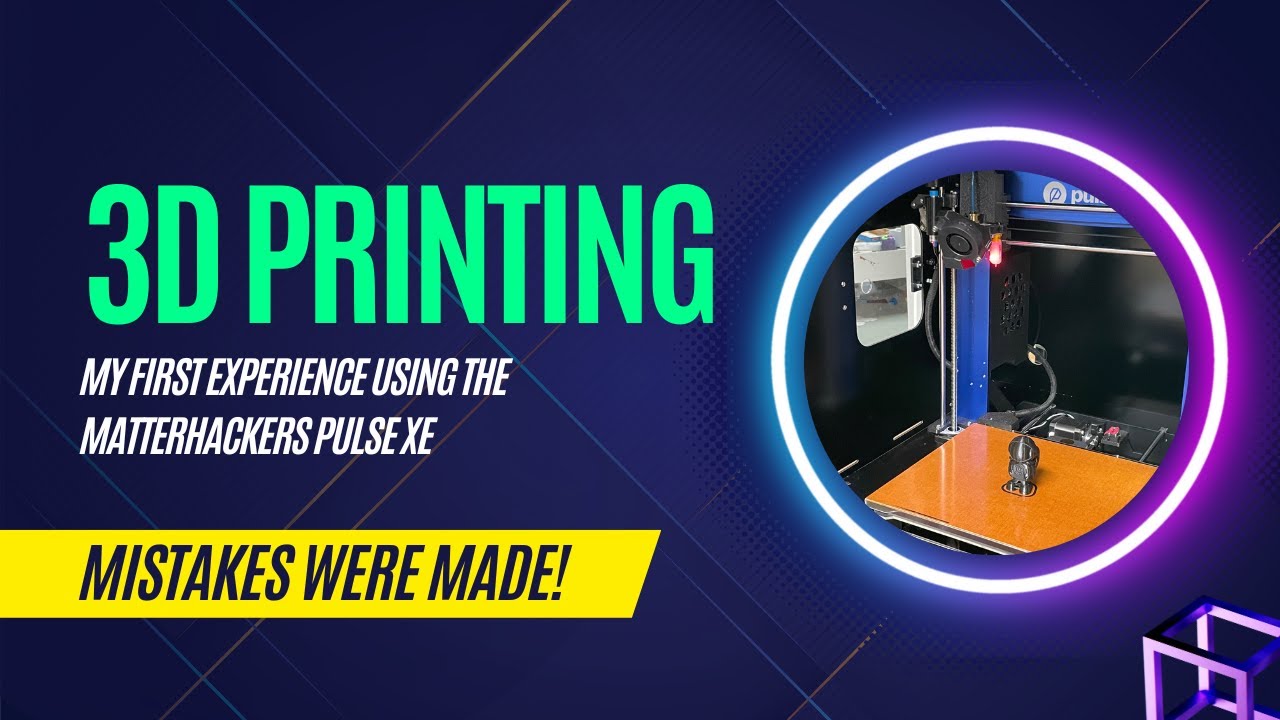The image features a dark blue background adorned with light blue and brown lines forming an intricate pattern that evokes the appearance of pixelated squares and geometric shapes. Prominently displayed in light green capital letters is the title "3D PRINTING." Below the title, in much smaller white capital letters, a subtitle reads, "My First Experience Using the MatterHackers Pulse XE." To the bottom of the image, there is a diagonally cut gray box with dark blue capital letters inside that exclaims, "MISTAKES WERE MADE!"

To the right side of the background, a glowing neon light circle highlights a photograph of a machine. The machine includes a visible motor and is accompanied by a mirror on one side and a flexible hose or cable. Everything is set upon a wooden surface. Further in the background, a TV screen can be seen, adding to the technological ambiance of the image.